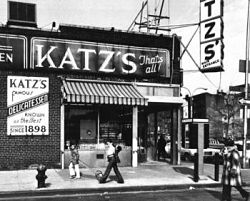The photograph is a striking black and white image capturing a slice of urban life from the past, possibly the 1930s, 40s, or 50s, set in what looks like old Philadelphia. The central focus is a single-story brick building marked prominently with a store sign that reads "Katz's, that's all!" in large white letters on a dark background. This storefront features a glass facade underneath a striped awning. In the foreground, a fire hydrant dating back to 1898 stands on the sidewalk, suggesting the long-standing history of the location. 

A small crowd of people, including children and adults dressed in mid-20th-century clothing, leisurely traverse the sidewalk. One child wears dark pants with a light shirt, while another sports a dark shirt and light pants. Near the scene, a person in a plaid shirt or coat and black pants meanders, while another figure dressed entirely in black lingers in the background. 

Additionally, there is an old automobile parked on the right side of the road, which is paved in black. The surrounding area features various old buildings, indicating a dense urban environment. Details such as a light pole, a possible stoplight, and a phone booth add to the cityscape's complexity. Despite being devoid of color, the photograph's intricate elements vividly evoke the era and locale it represents.